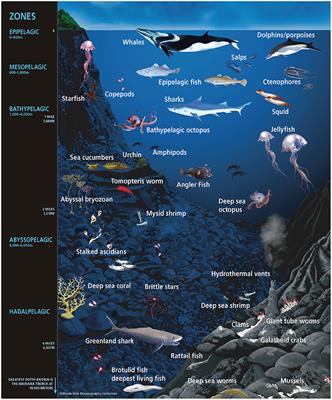The image is a detailed, vertically rectangular underwater poster that serves as a cross-sectional diagram of the ocean. The background features varying shades of dark blue, depicting different ocean depths, with the top showcasing a line representing the water surface under a slightly lighter blue sky. The poster is labeled to identify various marine animals at different oceanic zones.

At the topmost layer, called the epipelagic zone, whales and dolphins can be seen near the water's surface. Descending into the mesopelagic zone, a variety of fish are illustrated, swimming among submerged plants. Further down in the bathypelagic zone, jellyfish, squid, and deep-sea creatures such as anglerfish and octopuses populate the scene.

The poster also marks specific ecological niches like hydrothermal vents surrounded by deep-sea shrimp, giant tube worms, and brittle stars. The bottommost layers feature creatures like the rat tail fish, deep-sea sharks, and mussels. On the left side of the poster, a vertical black band labels the different oceanic zones, such as the epipelagic, mesopelagic, and bathypelagic areas, providing a clear educational guide to the diverse marine life present at various depths.